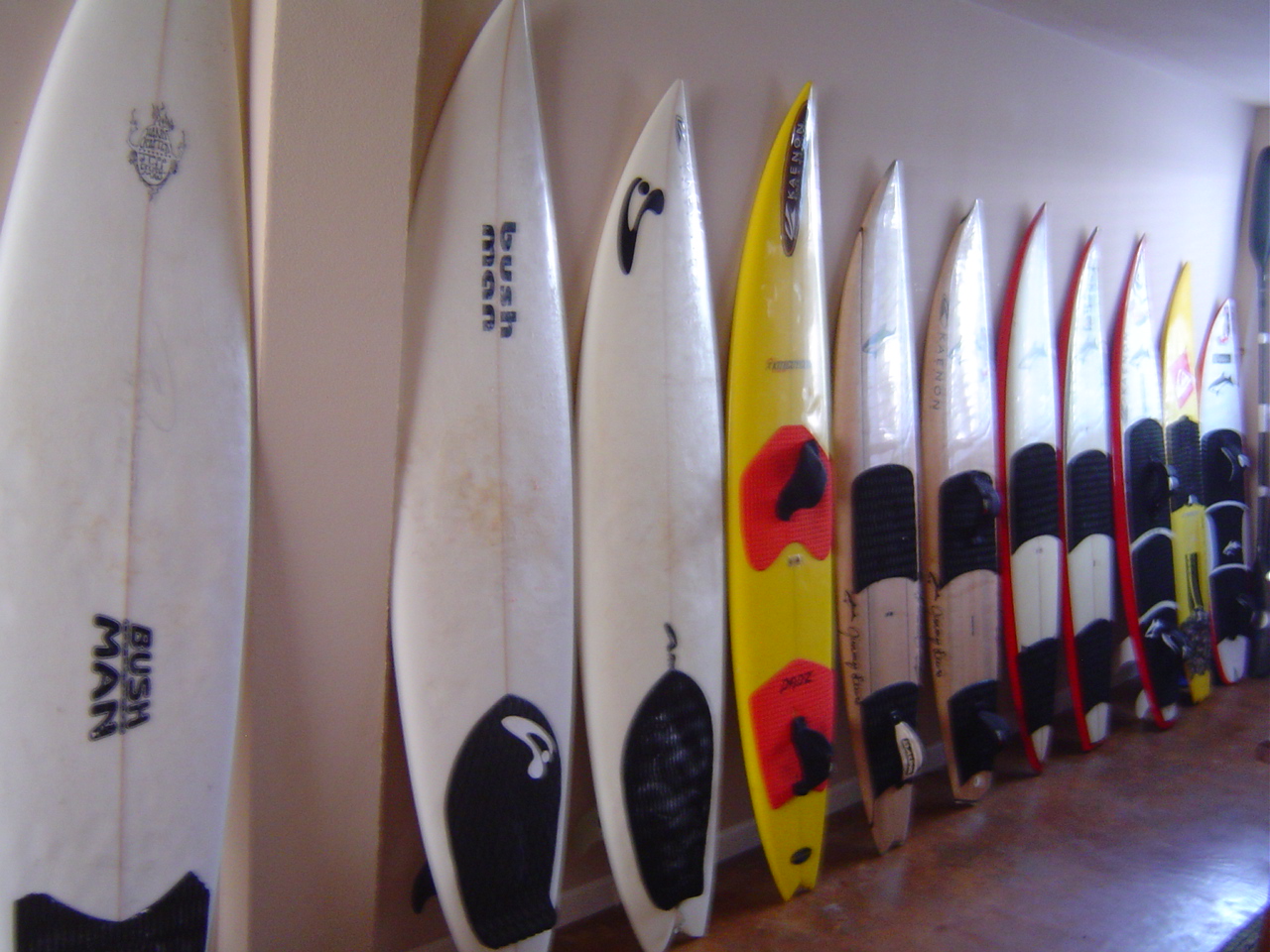Inside a large room with a polished brown concrete floor, an unfocused photograph reveals a collection of surfboards lined up vertically against a grayish-white wall. The surfboards are organized by size from left to right, with the longest on the left and the shortest on the far right. The first two on the left are Bushman surfboards, visibly used with some peeling paint. The majority of the surfboards are white with black lettering and symbols. Among them, a few stand out: near the middle is a bright yellow surfboard with orange and red details, and towards the right are additional yellow and white surfboards with red bottoms. In total, there are eleven surfboards, reflecting the room's lighting, some showing signs of wear.